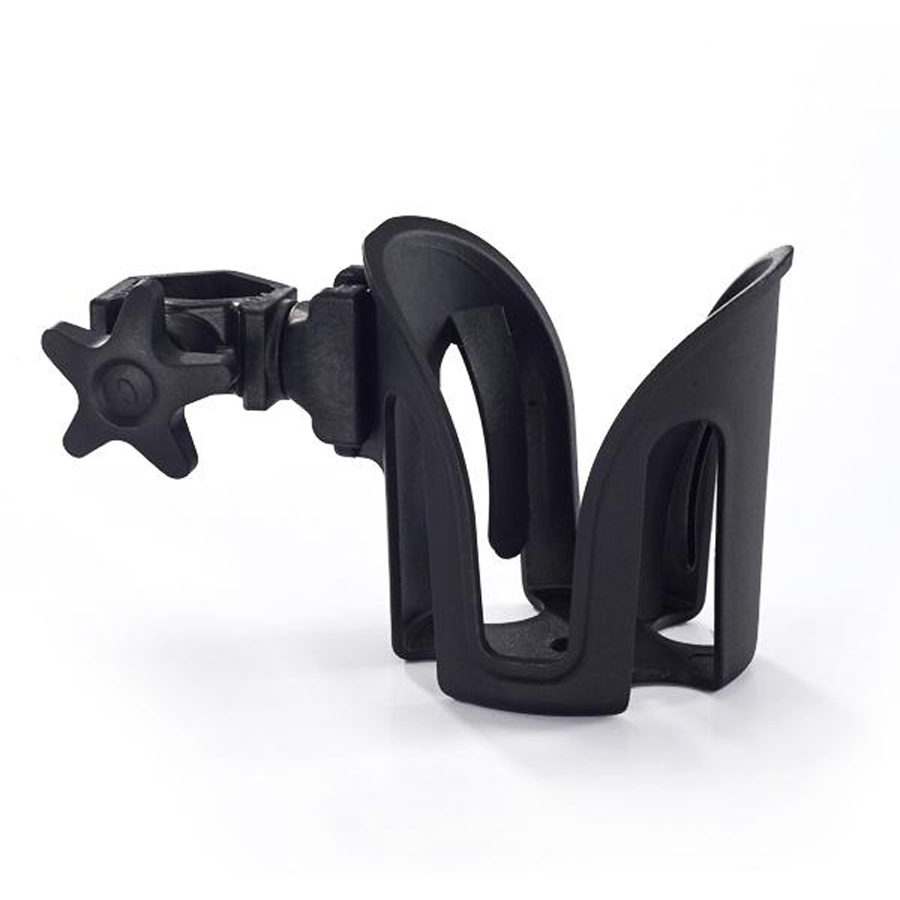The image showcases a well-made, black plastic cup holder designed for mounting, potentially on a bike or inside a car. The cup holder features a unique design with slats, likely included to reduce weight and improve aerodynamics. The holder itself has a structured, rounded shape with two edges at the top that curve outward, and four arms extending towards the middle, securing the cup in place. On the back, there is an adjustable circular opening equipped with a knob, resembling a hose tightener or a water faucet handle, which allows it to firmly attach to a surface like a pipe or a part of a vehicle. The background of the image is white, emphasizing the distinct features of this intriguing and functional piece of equipment.